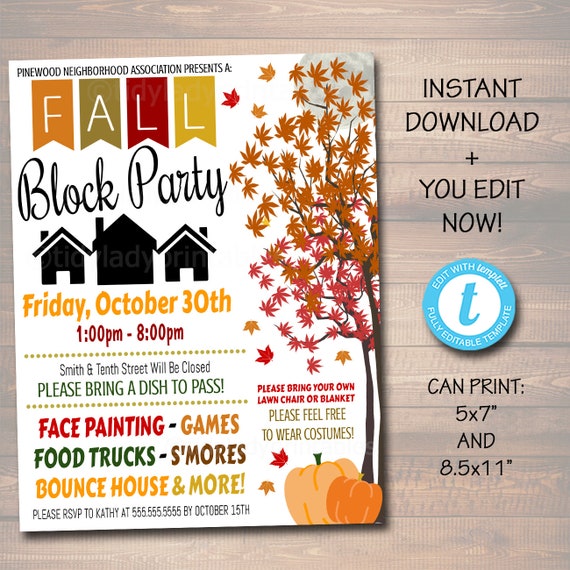The image is a computer-generated advertisement design for a magazine featuring an upcoming neighborhood block party. The design showcases a magazine prominently placed on the left against a slightly grayed-out wooden background. Beside the magazine, which has a pure white cover titled "Fall Block Party," are details that read, "Instant download plus you edit now. Can print: 5 by 7 inches and 8.5 by 11 inches." A circular disk with a 'T' in the center indicates, "Edit with template, fully editable template."

The magazine cover itself is rich with autumnal imagery. It features elegant title text at the top, reading "Fall Block Party." Central to the cover design are vibrant visuals of a tree with thin branches adorned with orange, pink, and red leaves, some of which appear to be blowing away. At the base of the tree is a picturesque arrangement of two pumpkins—one large and one medium-sized—adding to the seasonal theme.

Additional text on the cover announces, "Pinewood Neighborhood Association presents: Fall Block Party," followed by the event's details: "Friday, October 30th, 1 pm to 8 pm. Smith and 10th Street will be closed. Please bring a dish to pass. Face painting, games, food trucks, s'mores, bounce house, and more. Please bring your own lawn chair or blanket. RSVP Cathy by October 15th." Further enhancing the invitation are drawings of houses under the text "Block Party," adding a charming, community-centric touch.